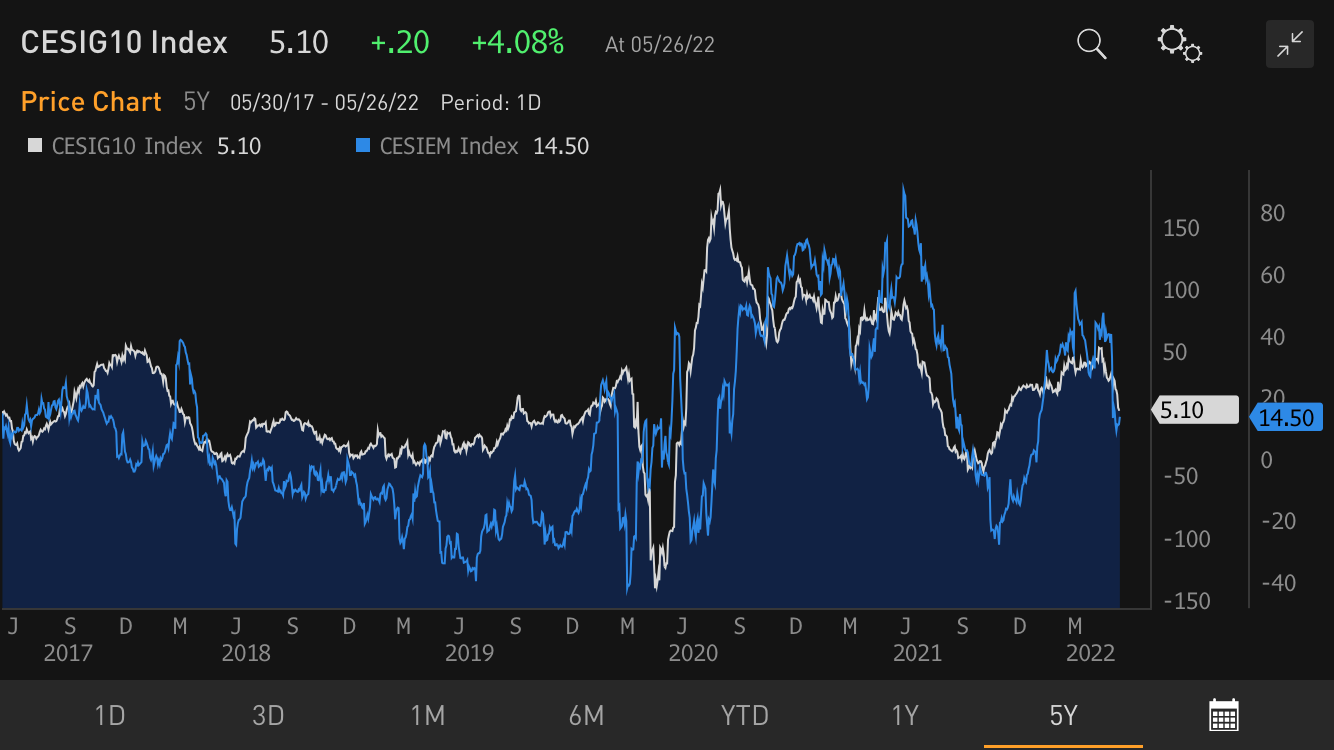In the provided image, there's a detailed price chart with a visual resemblance to an EKG graph. The chart features two prominent lines: one in vibrant blue and the other in vibrant white, with both lines fluctuating up and down across the timeline. At a certain point, one of the lines dips significantly.

To the right of the chart, there are two columns of numbers. The first column begins at 150 and prominently highlights 510. The second column starts at 80 and includes markings for 60 and 40, prominently highlighting 1450 in blue.

At the top of the chart, the SEGIG 10 index is displayed, indicating a span of five years. Key index values of 510 and 1450 are emphasized, corresponding to the highlighted numbers in the columns. Below the chart, there are selectable time ranges from one day up to one month, one year, and five years, providing various perspectives on the data.